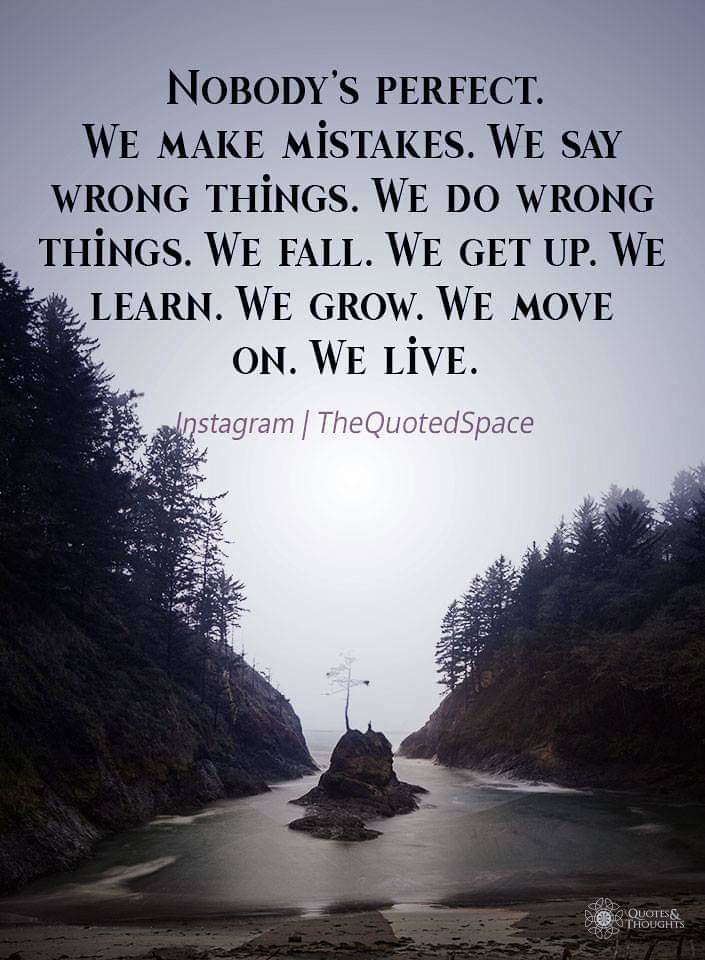The image is a motivational poster with an inspirational quote set against a natural landscape background. The scene captures a serene outdoor setting, likely during the day, featuring a sandy or dirt beach in the foreground that transitions into a body of water. The water is flanked by two large embankments or islands on either side, adorned with trees and foliage. In the center, there is a smaller land mass or hill, with larger hills and more trees extending to the left and right. The sky above is gray, adding a serene yet solemn atmosphere to the image.

At the top of this vertical rectangular image, the text reads: "Nobody's perfect. We make mistakes. We say wrong things. We do wrong things. We fall. We get up. We learn. We grow. We move on. We live." Below this primary text, in the center of the image, it states, "Instagram, the quoted space." Additionally, the bottom right corner of the image includes the phrase "quotes and thoughts."

The colors in the image are predominantly gray, black, purple, green, tan, and white, which contribute to the earthy and calming vibe of the scene. The style and setting of the image clearly align with that of an inspirational social media post intended to deliver a positive and motivational message.